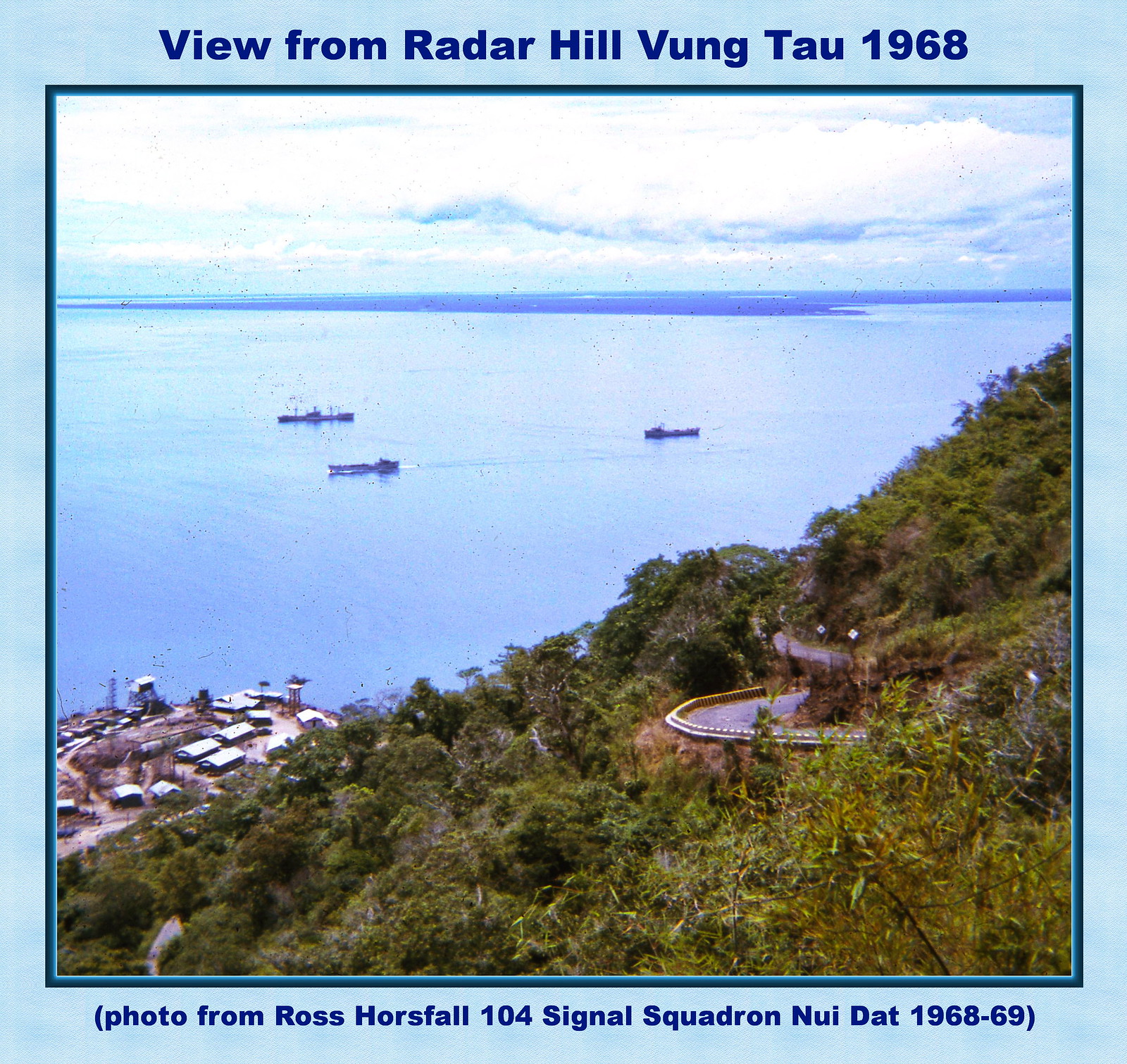This detailed image features a light blue border with text at the top reading, "View from Radar Hill, Vũng Tàu, 1968," and text at the bottom stating, "Photo from Ross Horsefall, 104 Signal Squadron, Nui Dat, 1968-69." The center of the image showcases a large body of water with three long, dark ships. Along the bottom left corner is a small town with several houses or structures, noticeable for their white roofs. To the right, a snaking road climbs up a tree-covered steep hillside. In the bottom right corner, the dense cluster of trees contains a visible fountain. The sky at the top of the image is mostly covered in clouds. The photograph captures an outdoor setting in Vietnam, with colors including light blue, dark blue, white, gray, green, yellow, and tan, suggesting it was taken in the middle of the day.